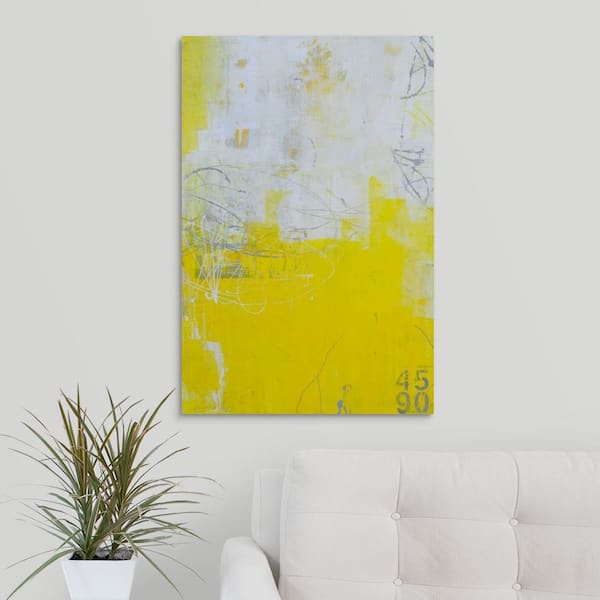The image showcases a minimalistic room, potentially a living room or an office, distinguished by its plain white wall. Dominating the lower right portion of the image is a partially visible white couch, featuring its back cushion and armrest. To the left of the couch stands a green plant with straight, spiky, brown, or green leaves, housed in a white pot. Above the couch and plant is an abstract, vertically-oriented painting. The painting is predominantly yellow in its lower half, transitioning to a dirty gray at the top. Black lines run across the canvas, adding to its streaky appearance. In the bottom right corner of the painting, faint numerical inscriptions are visible, with '45' above '90'. The overall color scheme of the photograph is minimal, limited to the white of the wall and couch, the green of the plant, and the striking yellow of the painting. No other objects or people are present in the image.